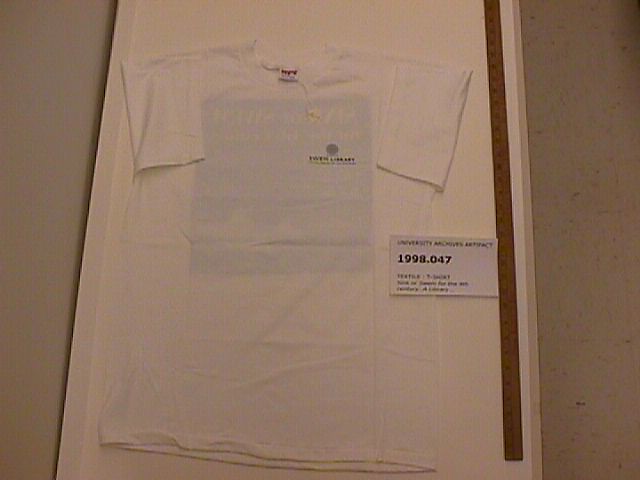The image depicts a white t-shirt neatly laid out, most likely on a cream-colored, speckled tile floor or behind a glass frame with a predominantly white background. The t-shirt exhibits both sleeves folded inward, giving it a well-arranged appearance. Accompanying the shirt is a yardstick or large measuring tape positioned along its left side, providing scale. A significant detail is the presence of a white cardboard paper or label, overlapping one edge of the shirt near the measuring tape. This label prominently displays the numbers "1998.047" in black text. The image quality is quite grainy and blurred, making other elements difficult to discern, including additional smaller text on the label. There's also a hint of additional design or text faintly visible through the t-shirt material. Overall, the image suggests that the shirt might be an artifact or collectible item, with the label providing an identifying code.